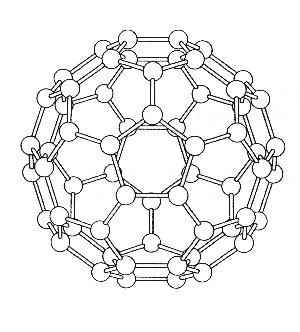This black and white computer-generated image portrays a complex molecular structure, with no background or frame. At its core, the design features a pentagon-like arrangement surrounded by approximately five concentric circles, each layer consisting of smaller spherical elements interconnected by thin rods. The central circle includes about six spheres, extending radially outward to larger circles, forming a spherical, lattice-like formation reminiscent of kinetic kids' toys from the early 2000s, which could collapse and expand. The overall structure gives the impression of a giant, intricate ball composed of interconnected smaller spheres.